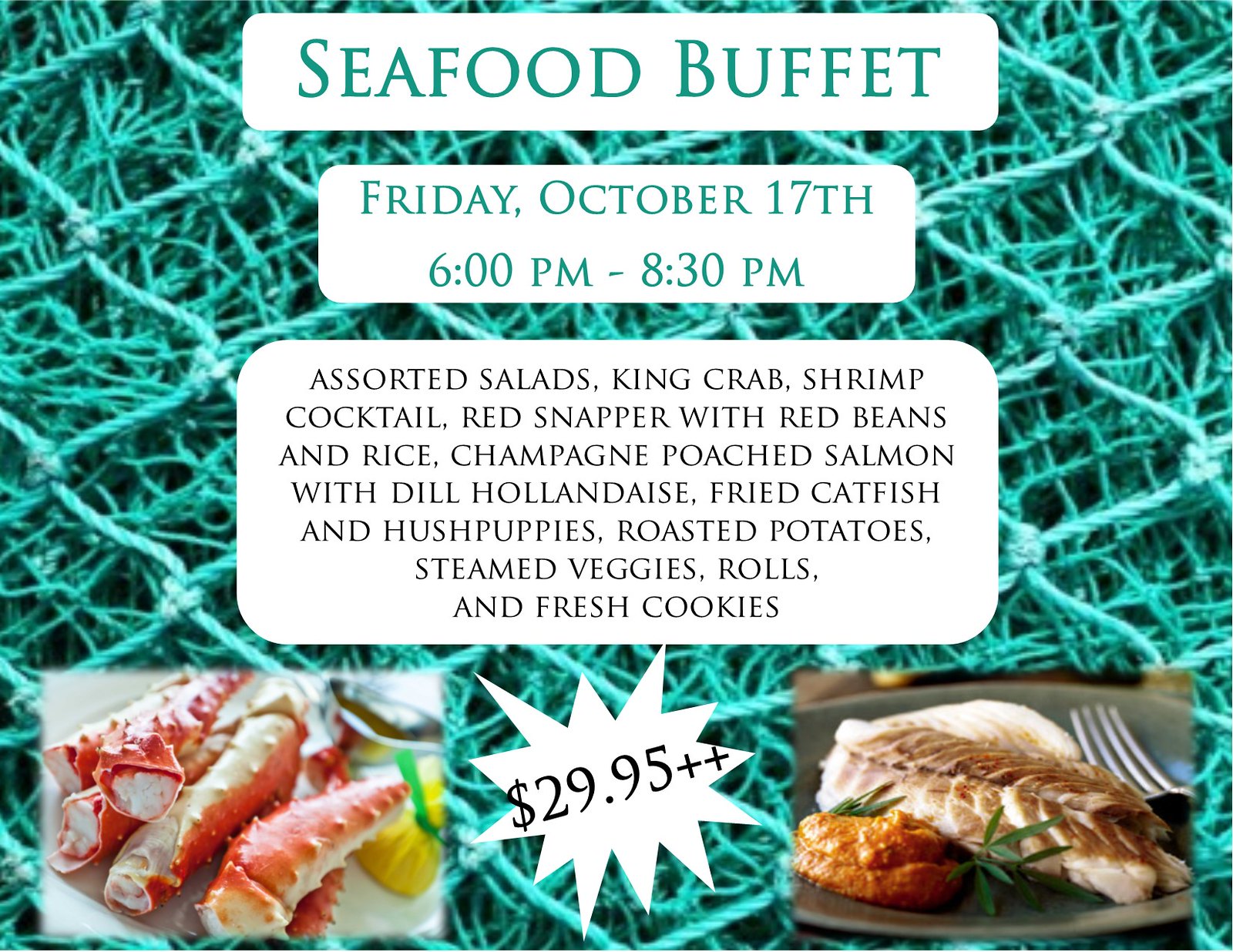The advertisement features a seafood buffet set against a light green to teal background, resembling interconnected strands of rope arranged in a chain-link pattern. Smaller strands, possibly hay-like in thickness, crisscross randomly throughout the background, adding texture. This intricately textured backdrop highlights several prominently displayed rounded white rectangles containing event details and food descriptions. At the top, bold green text announces the "Seafood Buffet," followed by another rectangle detailing the date and time: "Friday, October 17th, 6 p.m. to 8:30 p.m." Below this, a larger white rectangle with black text elaborates on the menu, listing items such as Assorted Salads, King Crab, Shrimp Cocktail, Red Snapper with Red Beans and Rice, Champagne Poached Salmon with Dill Hollandaise, Fried Catfish and Hushpuppies, Roasted Potatoes, Steamed Veggies, Rolls, and Fresh Cookies. Flanking the menu are two photographs; on the left, red crab legs, and on the right, a white and brown fish. Centered at the bottom, a multi-pointed starburst shape highlights the price, $29.95++, in bold black text.